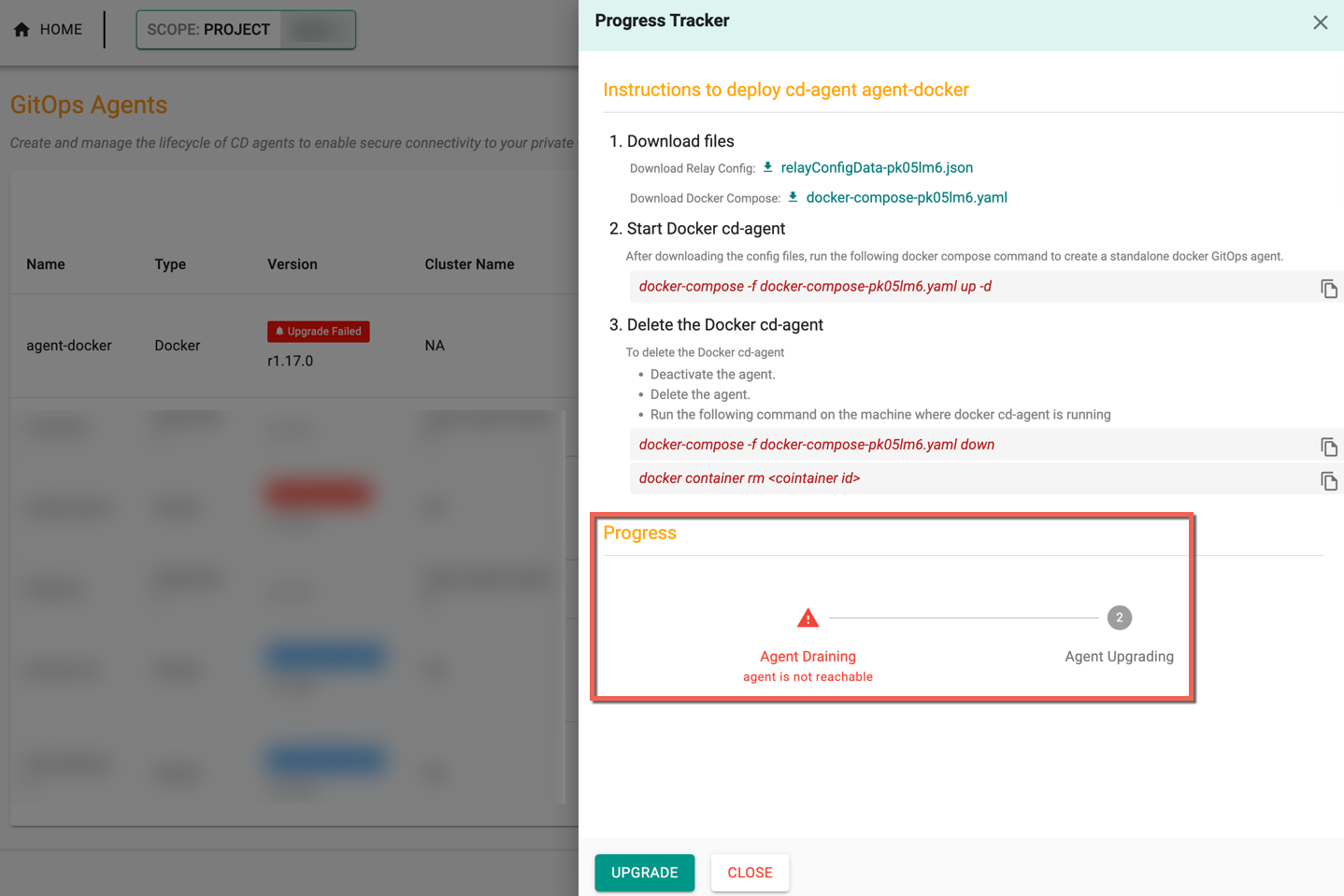The image showcases two distinct areas on a device screen. On the left side, the content is intentionally grayed out and muted, making details harder to discern. Despite this, various text elements are still visible, including "Get apps agents," "Agent Dacker," "Dacker," and "Upgrade failed." The lower portion of the left side is completely blurred for privacy reasons, with faint hints of red and blue colors visible.

Transitioning to the right side, the background is white, providing clearer visibility. At the top, a green rectangle contains the text "Progress Tracker." Below it, within a yellow background, are the instructions for deploying the "CD-agent" or "Agent-Dacker." The steps outlined are:

1. Download files
2. Start Docker CD agent
3. Delete Docker CD agent

Further down, there is a red-printed message, and at the bottom, a red-bordered progress rectangle states, "Agent driving agent is not reachable."